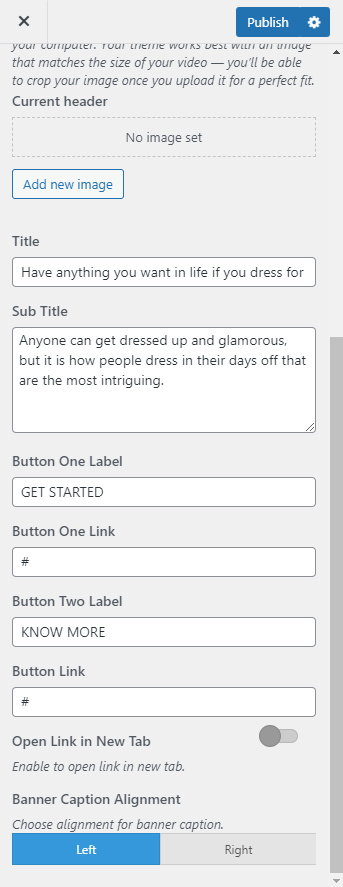This screenshot showcases an interface for editing a webpage or a blog post on a smartphone. 

At the very top, there is a close button represented by a small 'x', and to the right of it, a blue button with a white settings wheel icon and white text that reads "Publish."

Below these controls, partial header text is visible, followed by an interactive area outlined by a dotted line, labeled "New Image Set." Beneath this, there is a button labeled "Add New Image."

Further down, there is a space for a title, which begins with the text: "Have anything you want in life if you dress for." This is followed by a subtitle in its dedicated box: "Anyone can get dressed up in glamorous, but it is how people dress in their days off that are the most intriguing."

Additionally, there are four entry fields laid out from top to bottom. The first entry is:
1. Button 1 Label: "GET STARTED" (in uppercase)
2. Button 1 Link: A placeholder represented by a number symbol (#).

The second entry includes:
1. Button 2 Label: "NO MORE" (in uppercase)
2. Button 2 Link: Another placeholder indicated by a number symbol (#).

Further down, there are no additional entry boxes, followed by an option labeled "Open link in new tab." Next to this, a toggle switch is present, which is currently set to 'Off'. To the right of the toggle switch is the corresponding button.

Below this, the interface provides the option to "Enable to open link in new tab." 

Lastly, there's a section for "Banner Caption Alignment," where users can choose alignment for the banner caption. Two buttons are available here: a selected blue button labeled "Left" and an unselected gray button labeled "Right." 

This detailed description captures the various elements and options available in the screenshot, offering a comprehensive view of the interface.